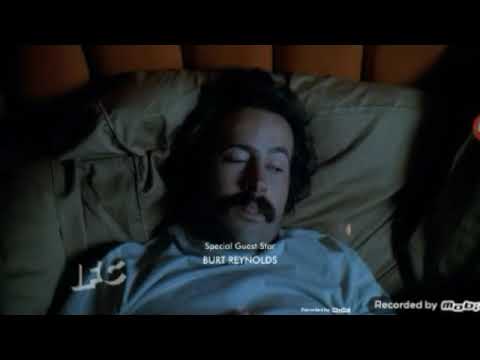The image is a screenshot from the TV show "My Name is Earl." It depicts a man with curly brown hair spread out across a beige pillowcase, laying on his back. His eyes are mostly closed, though one is slightly more open than the other, hinting that he is either half asleep or just waking up. He has a prominent dark brown mustache. He is wearing a light blue t-shirt.

The background shows a surface with what appears to be several vertical wooden columns. The lighting casts heavy shadows above him. The image is cropped with black rectangular bars at both the top and bottom.

In white text directly under his chin, it reads "special guest star Burt Reynolds." The bottom left corner of the image has "IFC" written in clear letters with a white shadowed outline. The bottom right corner partially shows "recorded by MOBA," though the text is cut off.